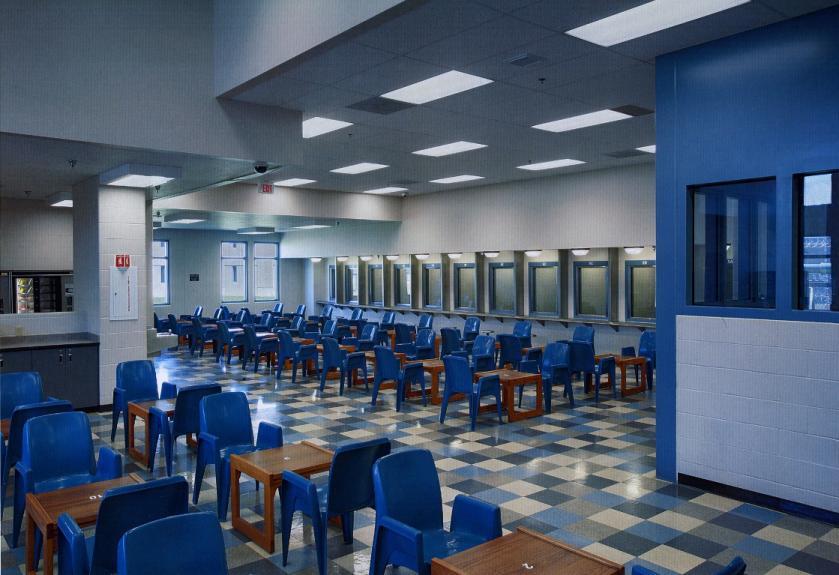The image depicts an interior scene, likely a waiting room or office with an arrangement that suggests it might be used for a cafeteria or even a DMV office. At the forefront, there are small desks paired with plastic chairs, arranged in rows facing each other, which could potentially serve for activities like card games or chess. The chairs are primarily blue, and the tables seem to be wooden with numbers on them.

In the middle of the image, a row of video panels can be observed. On the right side of the scene, there's a booth with windows. A fire extinguisher is mounted on a pillar to the left, which also appears to have a fire alarm. Overhead lighting is present, along with a camera positioned near an exit sign towards the back. The floor is a checkerboard pattern consisting of black, grey, white, and light blue tiles, which are reflective, adding to the overall brightness of the room. The back of the room features large windows that let in natural light, suggesting an overcast day outside. The color palette includes shades of blue, light bluish-gray, mahogany brown, white, black, and red.